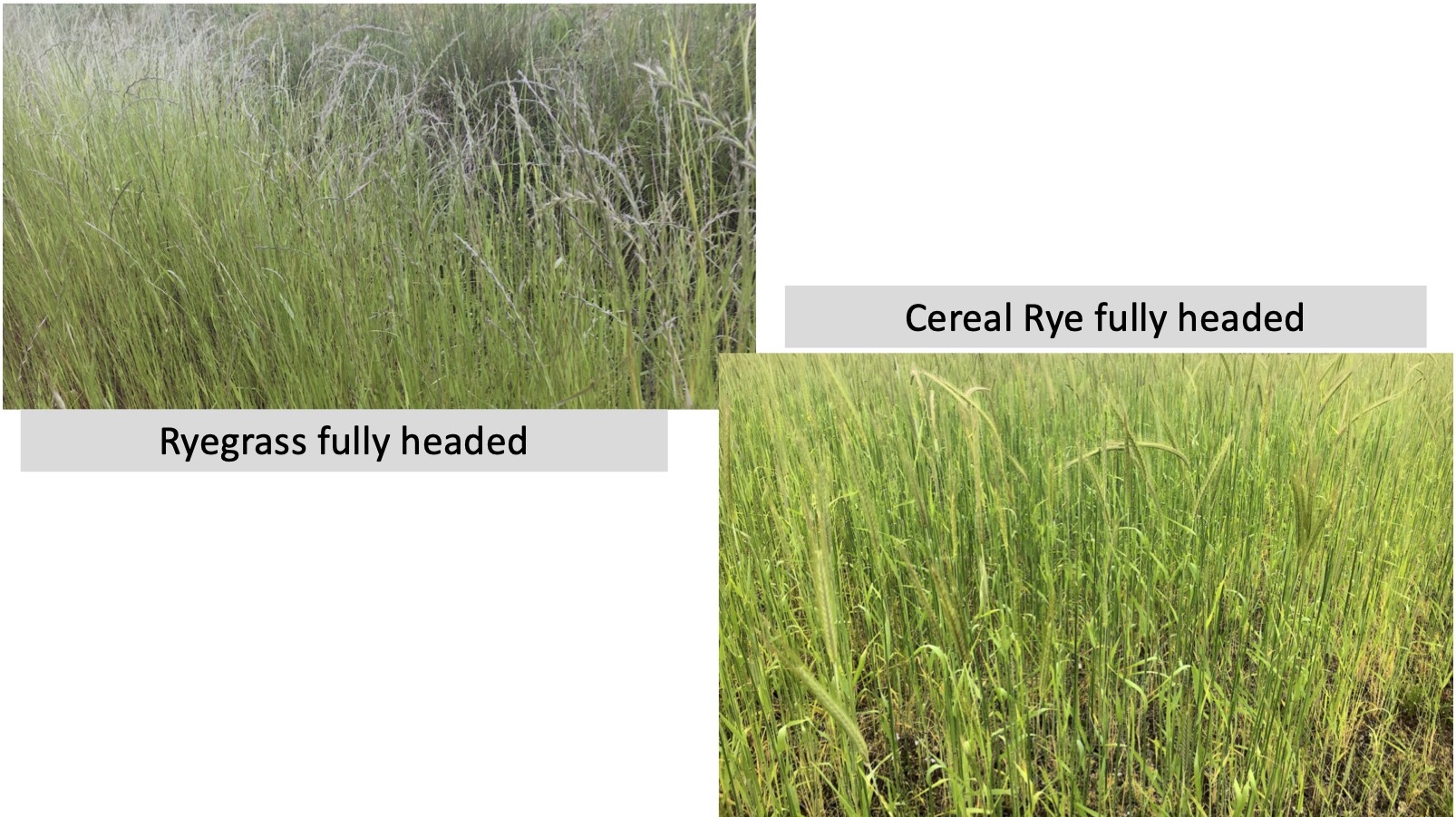The comparison image showcases two distinct types of grasses at their fully headed stages. The layout is devoid of a border and features two separated rectangular images diagonally aligned. In the top left corner, an image captioned "Ryegrass Fully Headed" displays green ryegrass with slightly brownish or grayish heads. This caption is presented in a gray box with black writing located below the image. In contrast, the bottom right corner of the image features "Cereal Rye Fully Headed," with its corresponding picture showing green cereal rye growing against a brown ground. This caption is also displayed in a gray box with black writing, situated above the image. The background of the entire comparison is solid white, emphasizing the differences between the ryegrass and cereal rye at their respective fully headed stages.